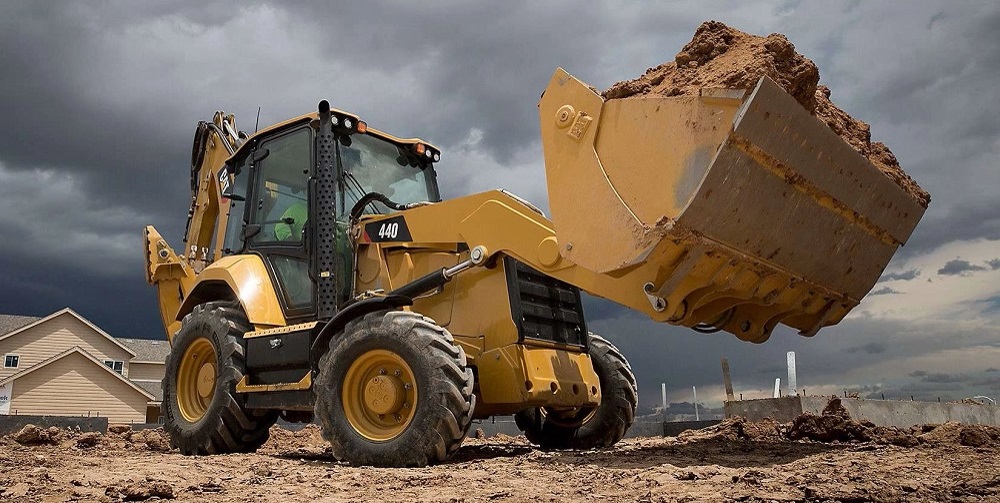In the photograph, a large yellow tractor sits prominently at the center of a construction site. The tractor, with its substantial four large tires and a spacious, windowed driver's cabin that looks capsule-like, holds an overflowing scoop of dirt lifted in the air at its front. There appears to be a driver seated inside, wearing a bright green jacket. The ground around the tractor is barren and brown, typical of an active construction zone. Behind the scene, a beige house with white windows and wood shingles stands, possibly under construction or recently built. Further in the distance, additional buildings and a pile of concrete are visible. The sky overhead is ominously dark and filled with gray clouds, suggesting an impending storm.